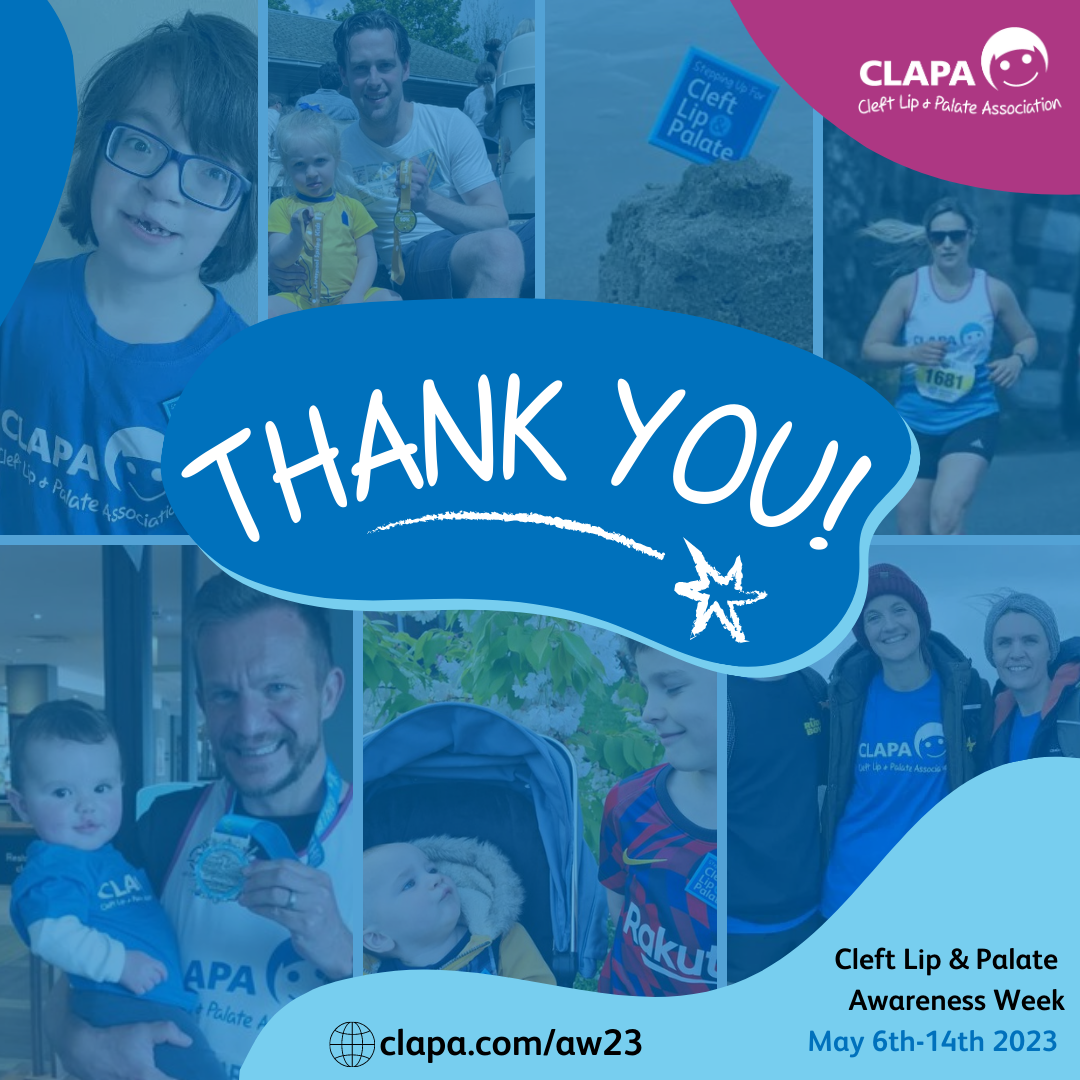This is a detailed poster for Cleft Lip and Palate Awareness Week, featuring a backdrop of various individuals, both children and adults, many of whom are smiling. The poster is primarily blue-tinted and prominently displays the words "Thank You" in the center, underlined with a star. 

In the top right corner, set within a violet semicircle, is the logo for CLAPA, the Cleft Lip and Palate Association. The logo includes a stylized child’s face with white hair, eyes, and mouth, alongside the text "Cleft Lip and Palate Association" in white.

The collage of images behind the central "Thank You" message includes:
- A child wearing blue glasses and a blue shirt, smiling.
- Another child in a yellow shirt next to a man with a white shirt and gray pants. The background shows several individuals in white shirts.
- An adult woman runner wearing a white and blue tank top with the number 1681, paired with black shorts.
- A small child in a blue shirt, white undershirt, and blue pants with short brown hair.
- An individual displaying an award, smiling, dressed in a white top with a black undershirt.
- Two children interacting: one in a yellow jacket sitting in a stroller and another in a sports jersey with red, blue, and partially obscured letters ("R-A-K-U-T") and a Nike Swoosh.

At the bottom of the poster is the web address "clapa.com/AW23" accompanied by a symbol of a world. The lower right corner details the event, stating "Cleft Lip and Palate Awareness Week, May 6-14, 2023" in blue text.

Additionally, there are images of a woman with a red beanie smiling, wearing a blue t-shirt under a gray jacket with a backpack, and another woman next to her in a gray beanie, orange and black jacket, also with a blue t-shirt and backpack. The overall theme underscores support and celebration of individuals connected to CLAPA.